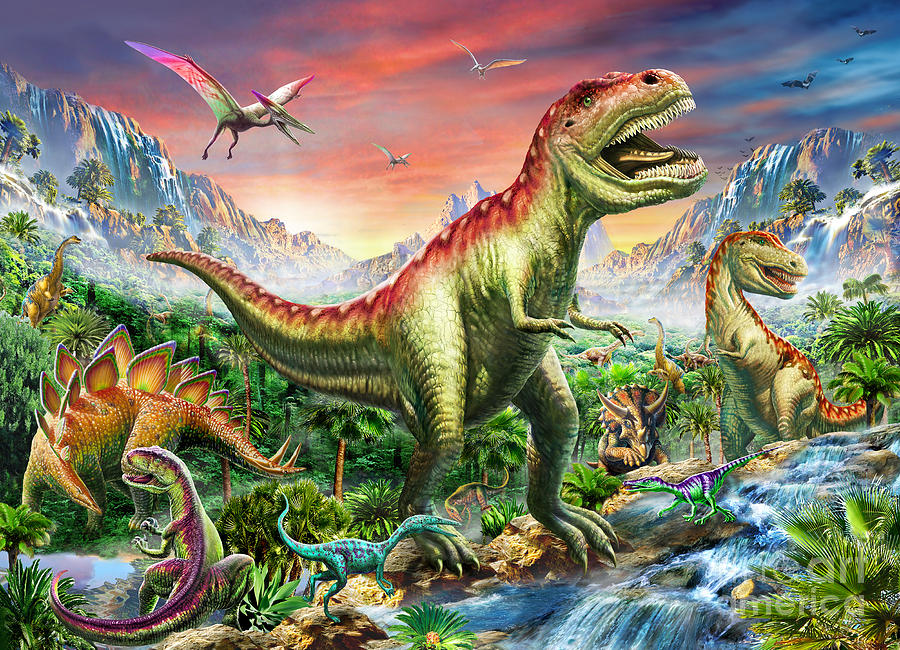This detailed illustration portrays a vibrant and imaginative prehistoric scene, set against a dramatic sky painted in shades of burgundy and blue, suggesting either dawn or dusk. Dominating the center of the image is a large T-Rex, its mouth agape to reveal rows of sharp teeth. Surrounding it is a multitude of vividly colored dinosaurs varying in size and species. A brontosaurus and a Triceratops can be seen among the mix, alongside Stegosaurus and other smaller, lizard-like dinosaurs dispersed across the terrain. Some dinosaurs sport imaginative color patterns, such as neon green with burgundy polka dots, or green with a purple stripe down the back, giving the scene a fantastical, almost video game-like quality.

In the foreground, a rushing stream cascades over rocks, flowing towards a tropical landscape rich with waterfalls, fog, and lush trees. Mountains and large rocky outcroppings rise in the background. Pterodactyls and other flying creatures soar through the air, adding to the dynamic atmosphere of the scene. Despite its prehistoric setting, there are artistic touches that bring a modern twist, making it a truly captivating image. A watermark labeled "Art America" is subtly placed in the lower right-hand corner, marking the artist's creation.